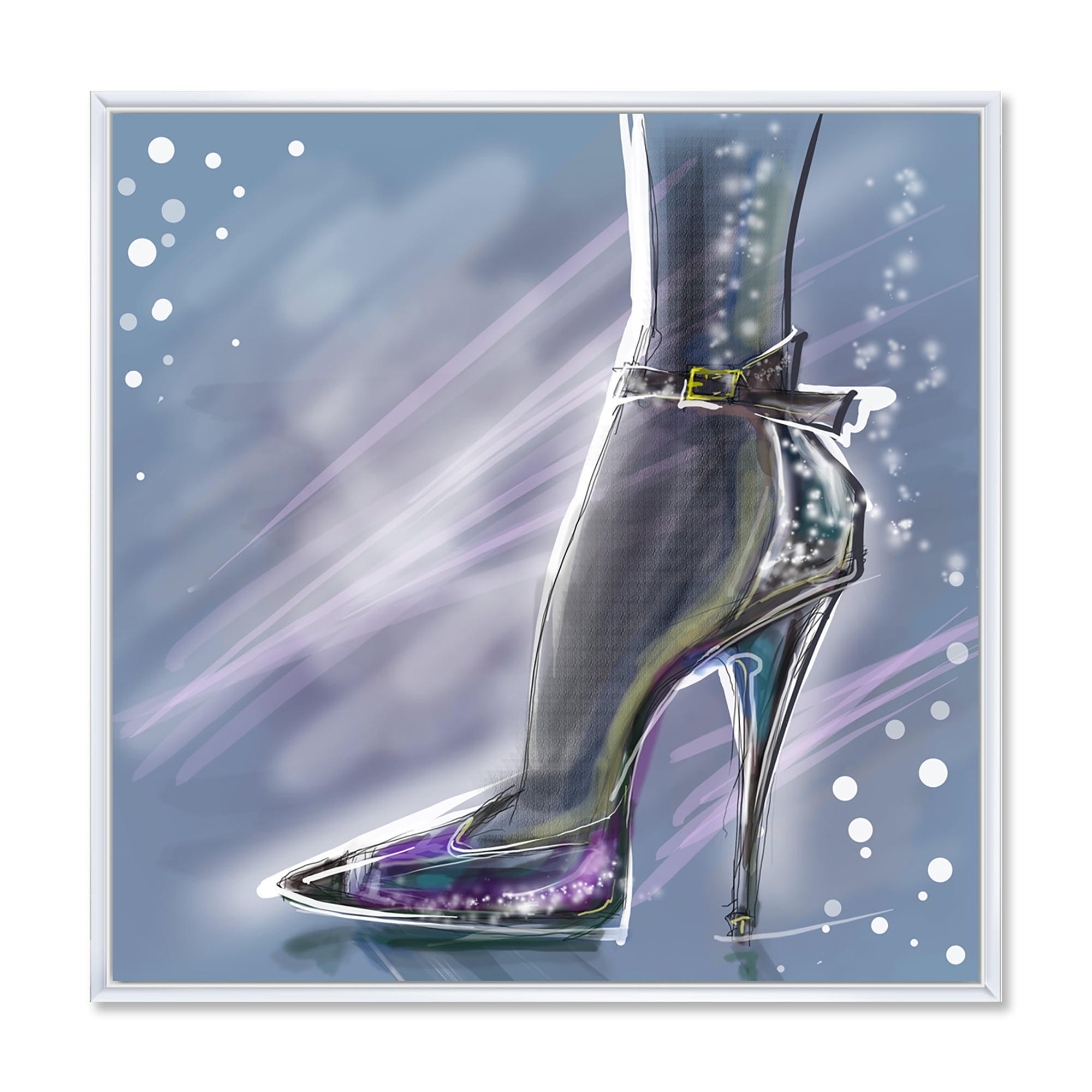The image is a digital artwork or painting featuring a woman's foot and lower leg from just above the ankle to the toes, clad in a very high-heeled shoe. The leg and foot are depicted in a gray or silver tone, giving a metallic, steel-like appearance. The shoe itself is high-heeled with a stiletto heel, exuding a jelly-like, semi-translucent quality. Reflective black and purple highlights accentuate the shoe, with the tip and heel in darker shades of black and purple. A gold buckle secures the ankle strap, adding a touch of elegance. The background is an abstract blend of blues, purples, and whites, adorned with numerous white dots, sparkles, and pink streaks, suggesting a bokeh effect. The overall aesthetic is sketchy and informal, with an emphasis on vibrant yet somewhat chaotic details surrounding the central figure.